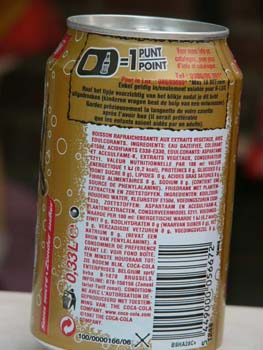The image depicts a prominently positioned aluminum can on a pristine white surface. The background, though intentionally blurred, subtly reveals hints of blacks, reds, whites, with delicate shadings of black, light pink, and a touch of purple. The can itself boasts a dark brown to gold gradient, providing a striking contrast against its white label. The label features bold, capital letters in a vivid red, accompanied by additional information contained within a slightly distorted rectangular box near the top, likely due to the curvature of the aluminum. The top and bottom rims of the can are exposed, displaying their natural metallic aluminum color.